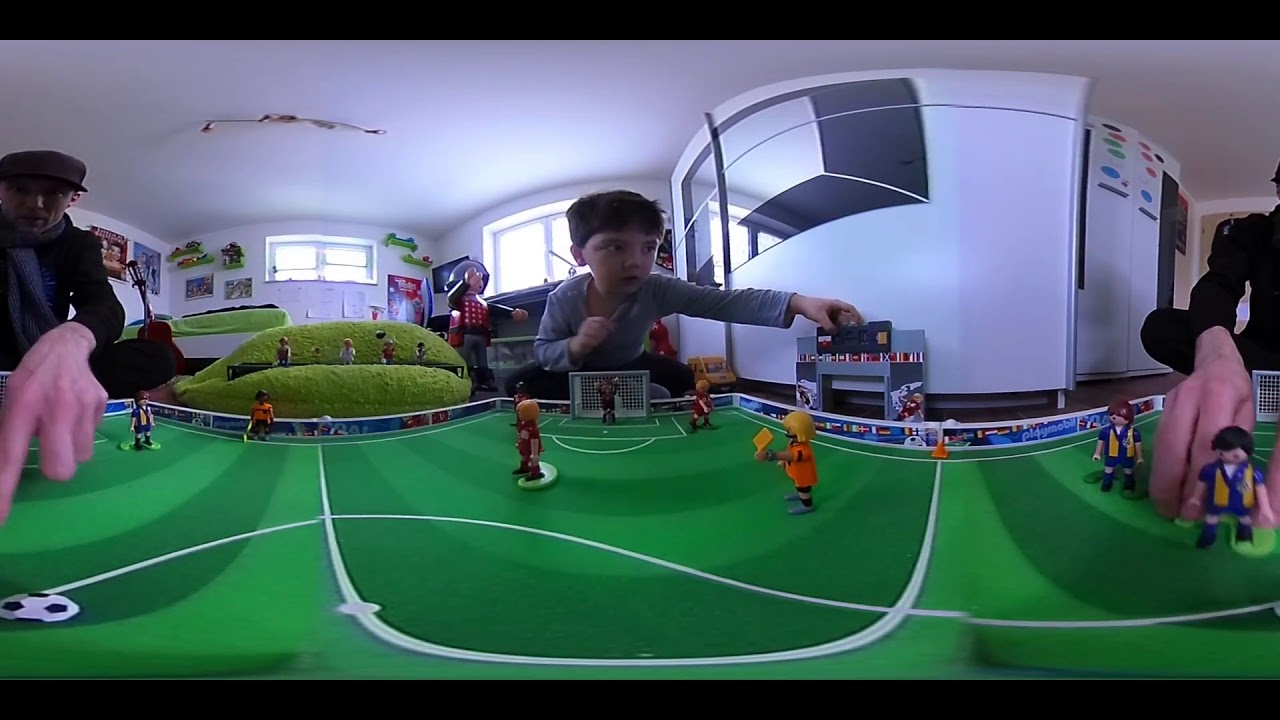The panoramic image captures a lively and detailed scene of children and an adult playing with a toy soccer field. The bottom half of the image prominently features the toy soccer field, adorned with light green and dark green stripes and white lines to indicate areas of play. At the center of this miniature field stands a plastic goal, behind which a figure in a black sports uniform is stationed. On the right side of the field, two toy figures donning yellow and blue sports jerseys, paired with blue shorts and black shoes, are visible. Centerfront, another toy figure in an orange uniform with gray shoes brandishes a yellow card. A black and white soccer ball rests in the bottom left corner of the field.

In the center of the image, a little boy with short brown hair, dressed in a gray long-sleeve shirt, can be seen grabbing a black object to his left. He is focused intently in that direction. Surrounding him, there are two people engaged in the game. The green playing area, with its distinct white lines, has a curvy shape adding depth to the scene. The room, presumably a game room, features white walls adorned with decorations and a white ceiling casting shadows. Other background elements include a light green mounded cushion and toy spectators on the benches watching the game. Additionally, a violin is discernible behind one of the figures, highlighting the room's multifunctional use.